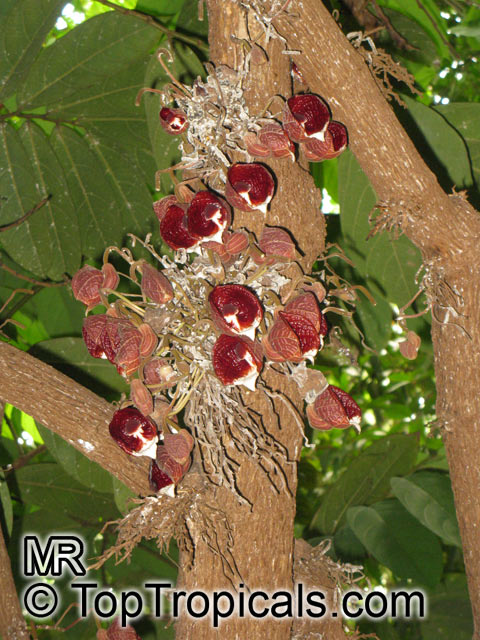A captivating rectangular nature photograph showcases a close-up view of a branch with striking red flower petals or possibly fruit. The branch, which is brown with white streaks, branches off to both the right and left, lying atop a bed of large, green leaves that span the entire background, suggesting a lush, outdoor setting. The image is slightly scattered with no centralized object, evoking a natural and untamed forest or garden scene. At the bottom of the image, in prominent text, is the website "MrTopTropicals.com." The diverse color palette includes various shades of green, brown, red, pink, and white, enhancing the natural beauty captured in the frame.